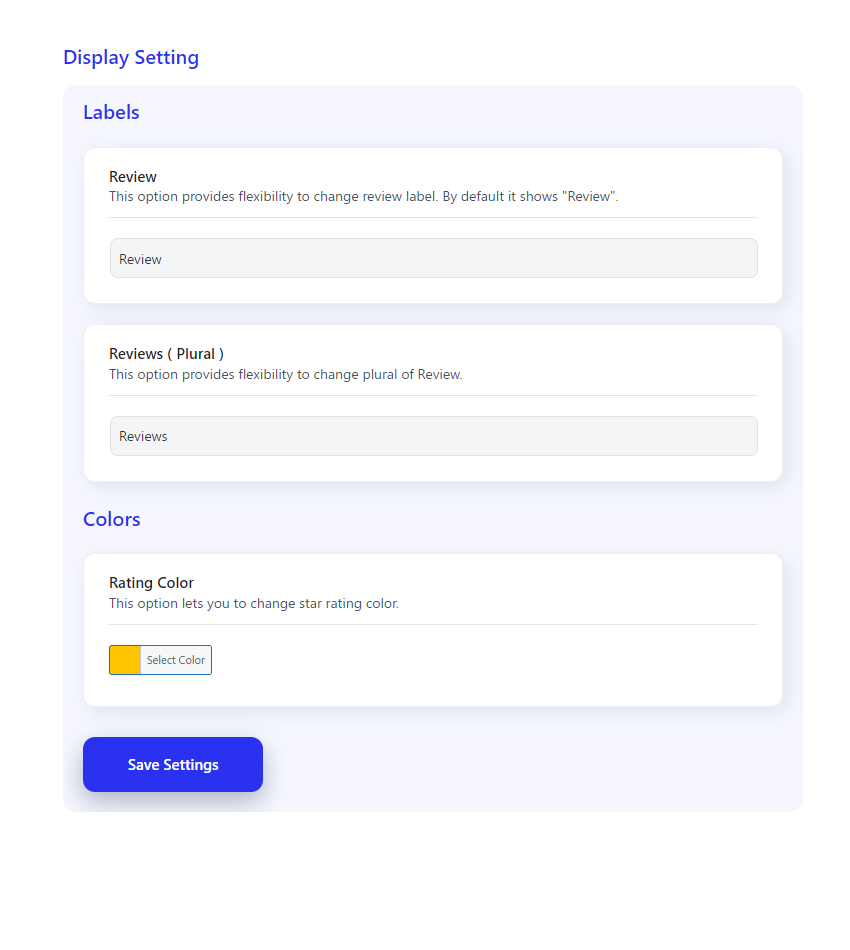Vertical screenshot of a smart device interface with a primarily white background. At the top-left corner, in blue text, it reads "Display Setting". Below that, against a gray background, there is a section titled "Labels" in blue. 

Within this section:
1. A white rectangular box displays the text "Review" in black with a less-bold font. 
2. Below the box, a descriptive line states, "This option provides flexibility to change the review label. By default, it shows 'Review'."

Following this label section:
- A thin black line separates a long gray box that also reads "Review".
- There is additional spacing before another white, rounded rectangular box, which contains the text "Review (plural)".
- Another description is provided: "This option provides flexibility to change the plural of 'Review'."
- A subsequent long gray box displays the text "Reviews".

Further down the interface:
- The section titled "Colors" is highlighted in blue.
- A white box reads "Rating Color" in dark black text, followed by, "This option lets you change the star rating color."
- A blue-outlined box labeled "Select Color" with the current selected color being orange.

At the bottom of the image:
- A blue, rounded button with white text reads "Save Settings".